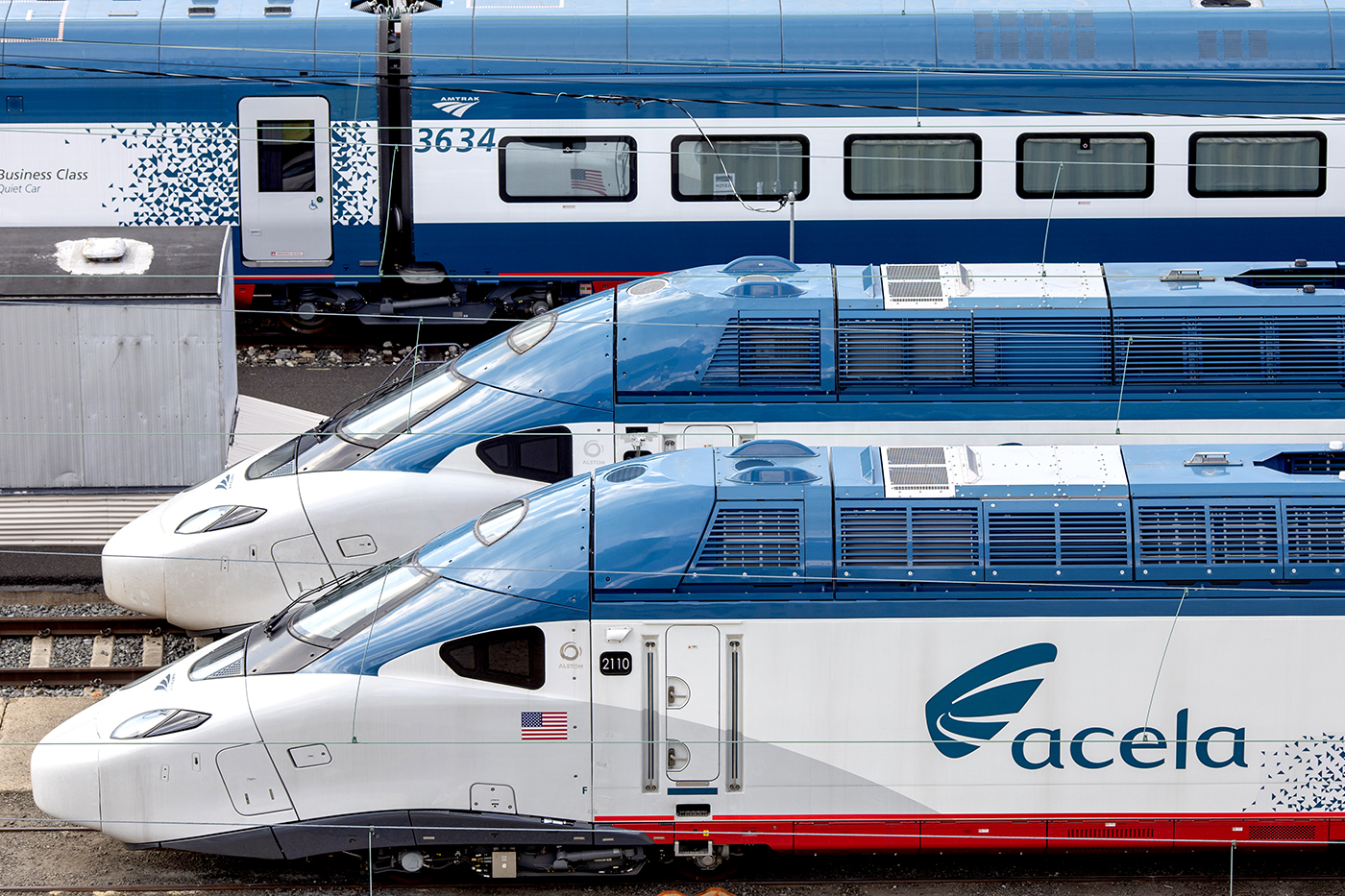The photograph, taken outdoors during the daytime, captures an array of three trains positioned on separate railway tracks from an elevated viewpoint. Dominating the foreground is the closest train, adorned with the name "A-C-E-L-A" prominently displayed on its side. This train features a distinctive color scheme with a bright blue upper section, a white midsection, and a red strip along the bottom. The front of the train slopes down into a sleek, narrow peak, and beneath the driver's window is an emblem of an American flag. Behind the forefront train lies a second, nearly identical engine, though its "A-C-E-L-A" labeling isn't visible. The train furthest from the viewer's perspective, likely where passengers sit, exhibits a blue top, white middle, and deep blue bottom, punctuated with the Amtrak logo and the number "3634." It also has prominent windows through which passengers can gaze. Additionally, the middle section is marked with the phrase "Business Class." Given the clarity of the shot and absence of motion blur, the trains appear to be stationary. The overall composition of the photo showcases a harmonious palette of blue, white, and red hues across all three trains, tying them together visually within the expansive outdoor setting.